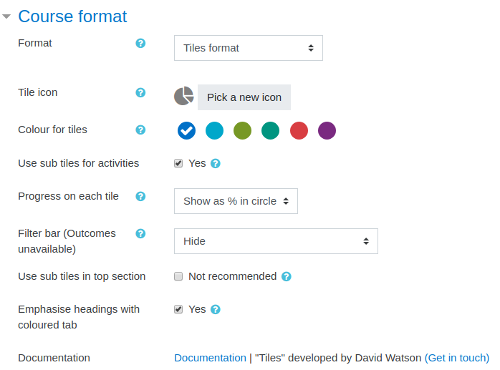Screenshot Description: 

The screenshot depicts a settings interface for configuring a course format, featuring a user-friendly drop-down menu labeled "Course Format" with the currently selected option being "Tiles Format". Beneath, there is a section titled "Tile Icon" displaying a pie chart graphic, where two segments of the pie are separated from the main circle, along with a prompt to "Pick a New Icon".

Further down, there's an option labeled "Color for Tiles", showcasing a selection of colors: blue, aqua, two shades of green, red, and purple, with blue currently chosen. The interface offers a toggle for using "Sub Tiles for Activities," which is activated, indicated by a checked "Yes" box. Under "Progress on Each Tile," users can choose from various display options; the selected choice is "Show as Percentage in Circle".

Additionally, a "Filter Bar Outcomes" feature is present but marked as "Unavailable" with a search bar, and "Hide" is the selected option. The settings also allow an option titled "Use Sub Tiles in Top Section," where a box labeled "Not Recommended" is unchecked. For emphasizing headings, the interface provides the "Emphasize Headings with Colored Tabs" option, which is enabled as shown by a checked "Yes" box.

At the bottom, there is a note about the "Documentation" and "Documentation Tiles" developed by "David Watson," including hyperlinks labeled "Get in Touch" and "Documentation".